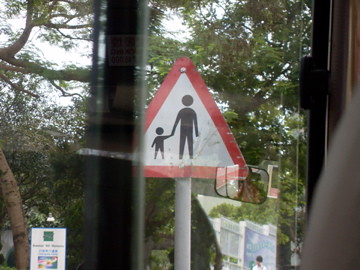A vibrant, small photo captures a scene taken through the window of a large vehicle, likely a bus, evidenced by the extensive glass and visible reflection of a driver and a rearview mirror. Dominating the foreground is a distinct school crossing sign, white and red, featuring the familiar black icons of an adult and child, the larger figure guiding the smaller one. The backdrop of the image is adorned with lush, green trees, adding a touch of nature to the urban context of the photograph.